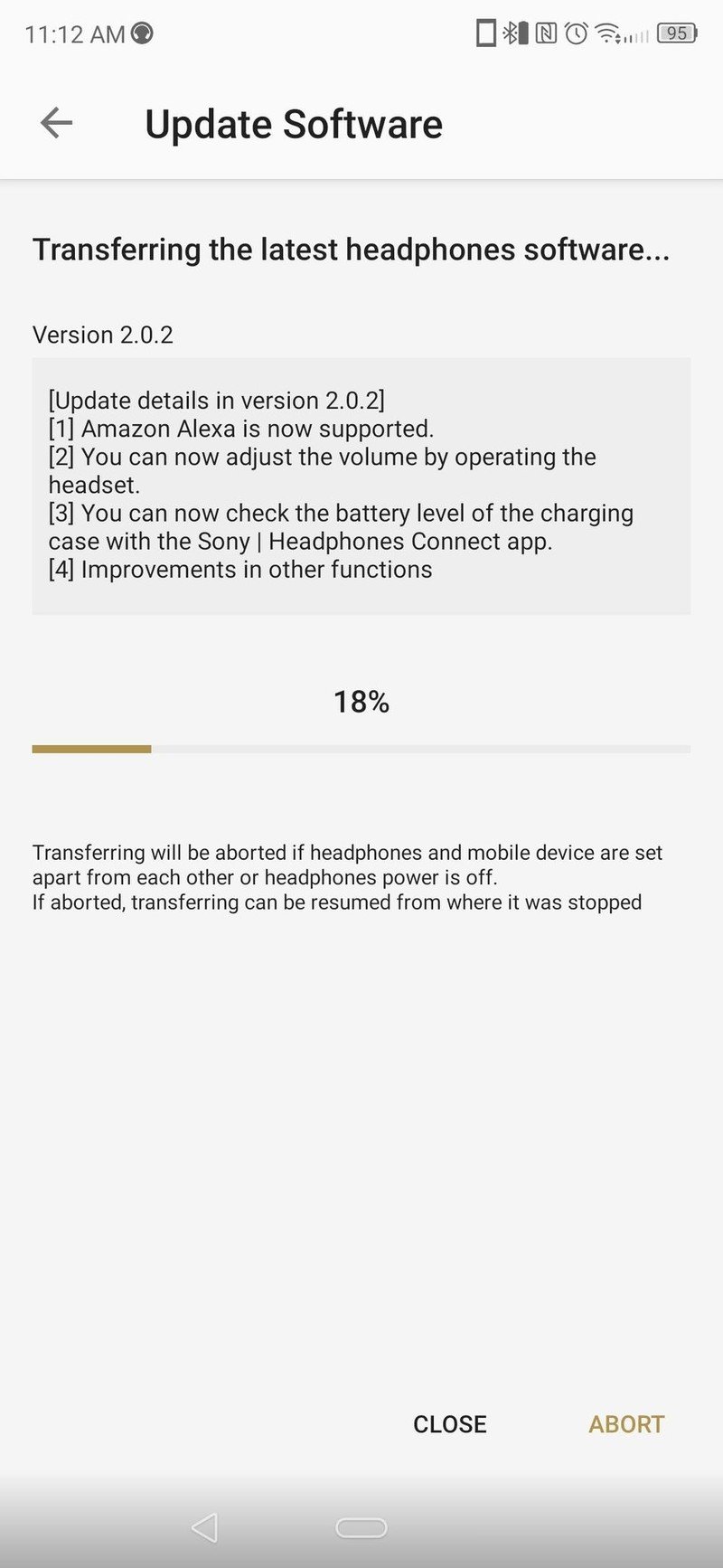The image shows a software update in progress on a mobile phone specifically for a pair of headphones. The time displayed at the top is 11:12 a.m., accompanied by a headphone icon. The screen header reads "Update Software" in bold black letters, with a back arrow on the left for navigation.

The main section indicates that the software update being transferred is version 2.2. Detailed update notes reveal: Amazon Alexa integration, the ability to adjust the volume directly via the headset, a feature to check the battery level of the charging case using the Sony Headphones Connect app, and several other functional improvements.

A progress bar depicting the update status is highlighted with a yellowish-brown color, showing 18% completion. The numerical value "18%" is written both above the progress bar and as part of the graphical indicator.

Further down, the screen includes a cautionary note in smaller black text: "Transferring will be aborted if headphones and mobile device are set apart from each other or if headphones power is off. If aborted, transferring can be resumed from where it was stopped."

At the bottom edge, two options are presented: "Close" in black letters and "Abort" in a yellowish-brown color. Finally, the bottom of the screen features a white triangle and a white oval shape, typical navigation icons of the mobile interface.